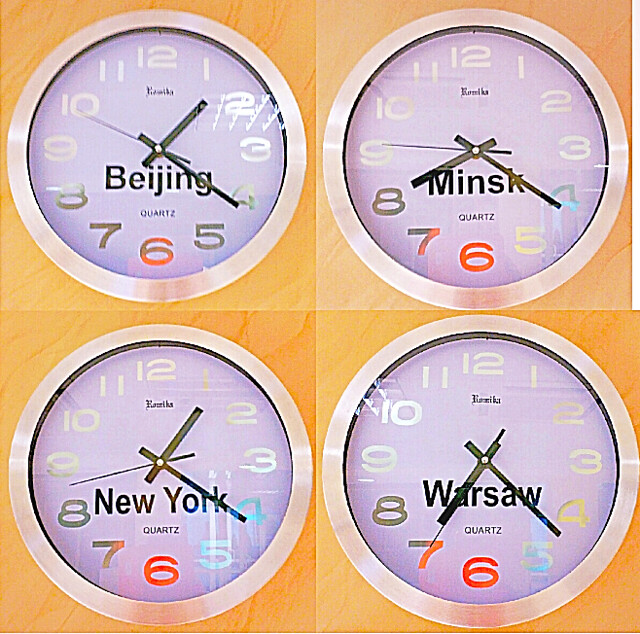This image showcases a set of four purple-faced quartz clocks, each indicating a different city's time, arranged in a 2x2 grid with visible wooden paneling in the background. Each clock is encircled by a stainless steel ring and features white numbers for 1, 2, 3, 9, 10, 11, and 12. The remaining numbers are colored distinctly based on each clock's city label. For Beijing, the numbers 4, 5, 7, and 8 are silver, with the 6 being partially silver and red. Minsk has a blue 4, white 5, red 6, a partially black and red 7, and a black 8. New York displays a blue 4, light blue 5, red 6, an orange and red 7 with a black top, and a black 8. Warsaw’s 4 is olive green, the 5 is partly white and blue, the 6 is red, the 7 is partly black and red, and the 8 is black. The displayed times are varied; the upper-left clock shows 1:20, the upper-right shows 8:20, the bottom-left again shows 1:20, and the bottom-right shows 7:23.